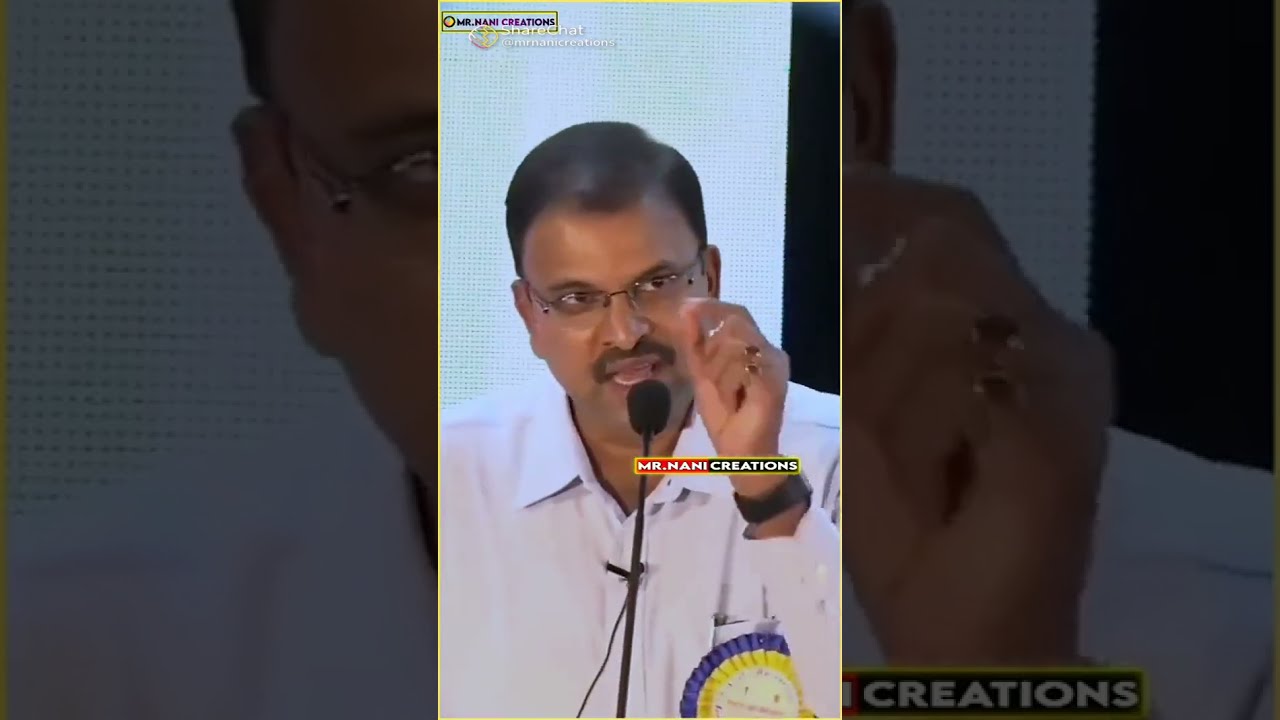A man with short, parted black hair, dark brown skin, and brown eyes is speaking into a long black microphone. He is wearing eyeglasses with top rims only, a white button-up shirt with what appears to be a pocket, and a black watch on his wrist. He has a mustache and two rings on his fingers. His hand is held up underneath his eye, with his index finger and thumb together in a point, emphasizing his speech. He displays a passionate and engaged demeanor. There is a circular medallion or ribbon pinned below his chest pocket, featuring a blue outer ring, a yellow middle, and a white inner circle. The background is white with black polka dots. The text "Mr. Nani Creations" is displayed both in front of him near his hand and at the top left corner, framed by yellow lines.